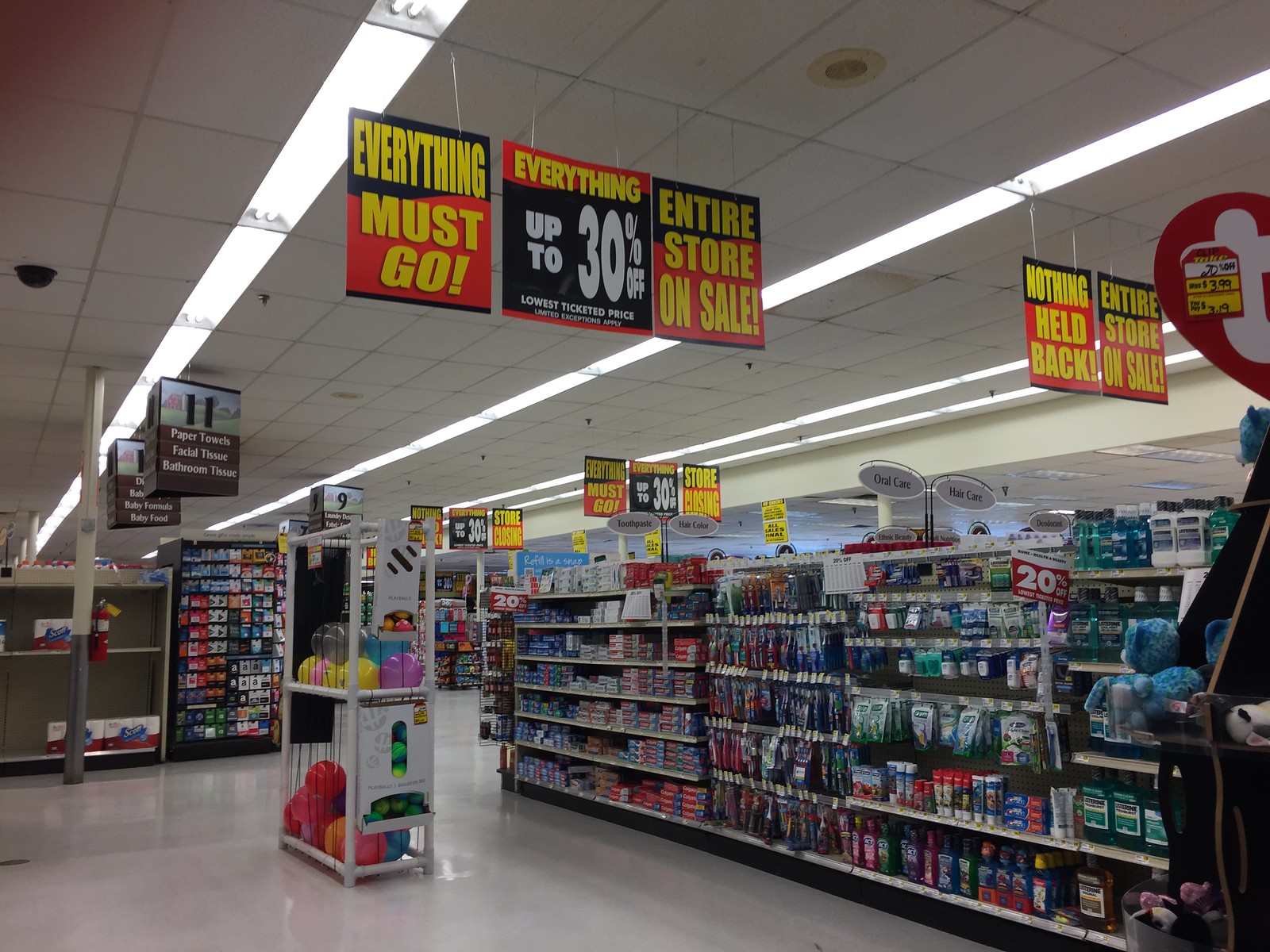The image depicts the interior of a store, showcasing a highly detailed and structured layout. The store's floor is composed of white, shiny tiles, contributing to a bright and clean ambiance, complemented by rectangular off-white ceiling panels adorned with fluorescent lighting arranged in rows from left to right.

In the foreground, a white shelf stands centrally, laden with a net filled with colorful balls—pink, blue, yellow, gray, and purple. To the right, more white shelves are visible, stocked with oral care items, including toothbrushes, mouthwash, and toothpaste. Adjacent aisles are partly obscured, though one sign visible in the background announces a hair care section.

On the left, shelves display Scot's toilet paper. Above these aisles, a series of prominent signs hang from the ceiling, emblazoned with bold promotional messages in yellow, red, black, and white backgrounds. The slogans "Everything Must Go," "Up to 30% Off," and "Nothing Held Back, Entire Store on Sale" are all featured in large, attention-grabbing letters, underscoring the store-wide sale. 

In the background, additional aisles and more identical orange, yellow, and black sale signs further indicate the store's comprehensive discount campaign. The overall scene is one of organized retail clearance, characterized by clearly demarcated sections and a variety of vividly colored promotional materials.